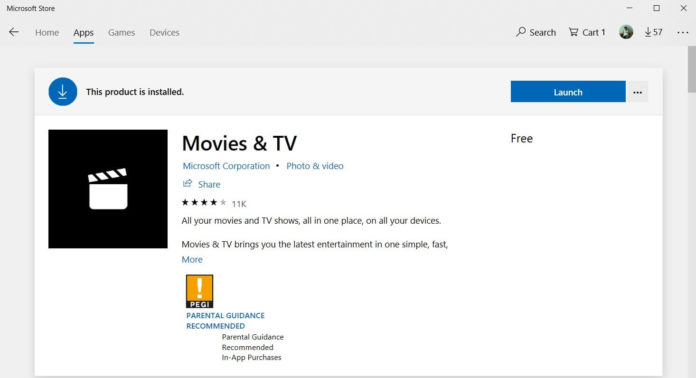This image depicts the interface of the Microsoft Store website. At the top left corner, the text "Microsoft Store" is prominently displayed. Directly beneath that, there is a left arrow icon followed by the word "Home." Adjacent to "Home," the menu options include "Apps," "Games," and "Devices," with "Apps" being highlighted by a blue underline, indicating the current section being viewed.

On the top right, there is a search icon accompanied by the word "Search." Next to the search icon, there is a shopping cart icon labeled "Part 1." Adjacent to the shopping cart, there is a circular icon that appears to be a profile picture placeholder, featuring a down arrow pointing to a line – potentially indicating a dropdown menu. Next to this profile circle, the number "577" is displayed.

Below the navigation bar, the rest of the screen is divided into sections. One section features a blue circle with a downward-pointing arrow next to the text "This product is installed." To the right of this, there is a blue "Launch" button followed by a vertical triple-dot menu (ellipsis) and a square icon.

Further down on the page, there is an image displaying a movie reel icon centered within a black square. Below this image, the text "Movies & TV" is shown, with "Microsoft Corporation" listed underneath as the provider, categorized under "Photo & Video." On the far right, the text "Free" is displayed along with some user ratings and additional information about the product.